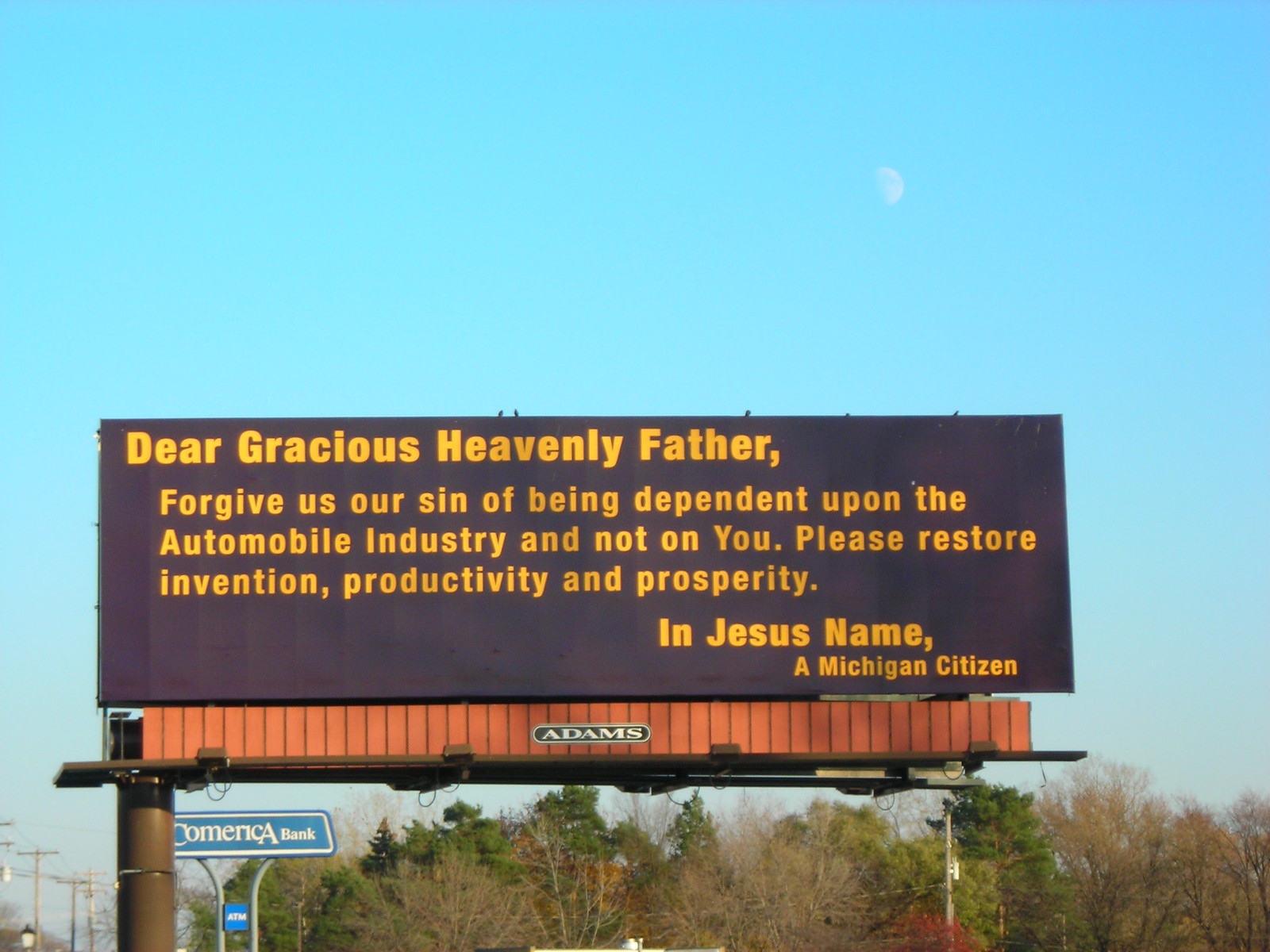This image captures a rectangular landscape outdoor billboard positioned on the side of a road against a backdrop of a light blue sky with a faintly visible moon in the upper right-hand quadrant. The billboard's dark brown surface prominently displays a religious message in mustard-yellow text: “Dear Gracious Heavenly Father, forgive us our sin of being dependent upon the automobile industry and not on you. Please restore invention, productivity, and prosperity. In Jesus' name, a Michigan citizen.” The opening and closing phrases, "Dear Gracious Heavenly Father" and "In Jesus' name," are in the largest font. Below the text, there's a long slim red rectangle featuring a cylindrical blue logo with the word "Adams" in white, indicating the billboard's manufacturer. The billboard is mounted on a thick brown pole located on its left side, leaving the right side unsupported. 

The scene below the billboard shows a mix of green evergreen trees and leafless deciduous branches, hinting at winter. On the left side of the image, there are utility poles extending into the background. In the bottom part of the image, nearer the right-hand side, a blue rectangular sign with white lettering reads "Comerica Bank," suggesting the presence of a bank nearby. The overall composition suggests a clear but cool day along the highway or roadside.